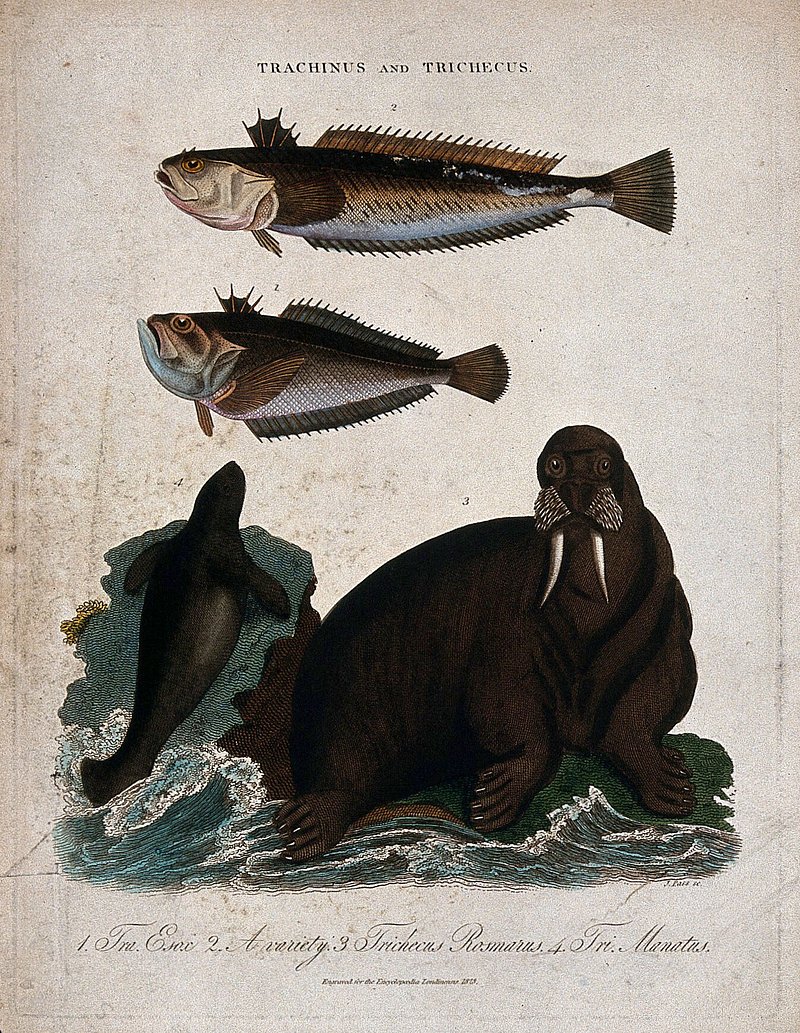The image presents a detailed, possibly hand-drawn or digitally created piece that appears faded and aged. At the top, there are two brownish fish labeled with the text "Trachinus" and "Trachicus," though the text is somewhat hard to read due to its small size. The top fish is long, while the one below it is shorter and stouter, both exhibiting light blue bodies and mouths. The fish are facing left. Below the fish, there are two images of walruses in water. One shows the back of a walrus swimming away, while the larger image, located nearby, depicts a walrus looking straight ahead. This walrus image reveals its two front flippers and a back leg. The overall color palette includes shades of dark brown, white, teal, light brown, green, and off-white, adding depth to the detailed and somewhat enigmatic composition.